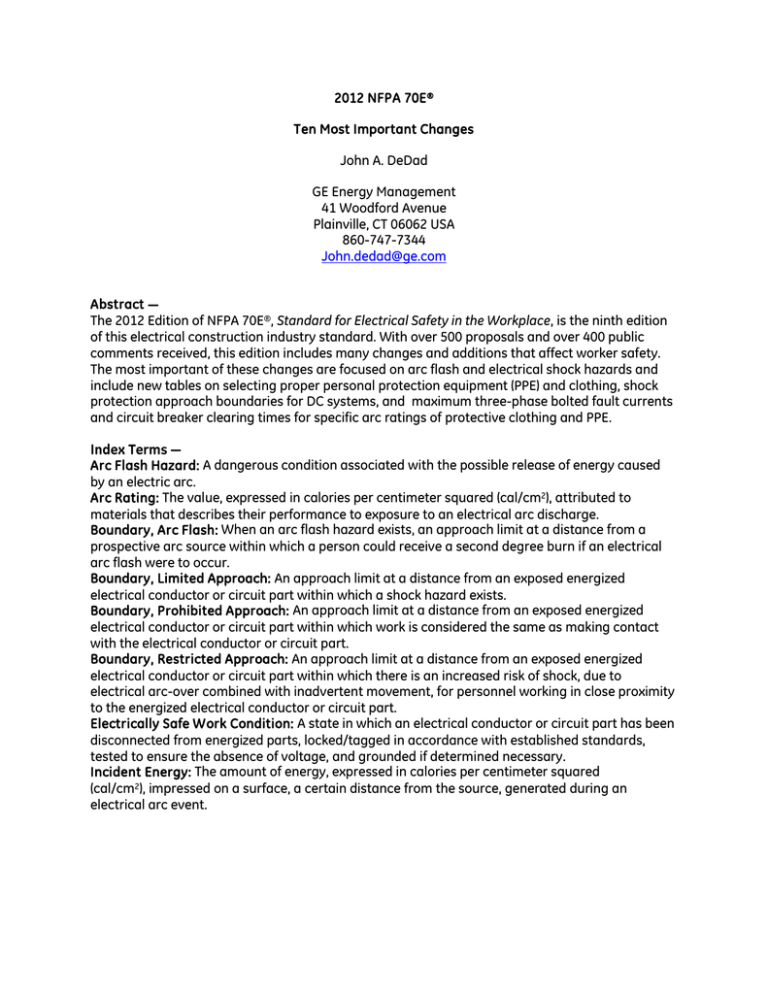The image features a clean, white background without any borders and primarily contains black text, interspersed with a blue web address. At the top, bold text reads "2012 NFPA 70E, 10 Most Important Changes" by John A. Dadad, GE Energy Management, 41 Woodford Avenue, Plainfield, CT. Below this heading, there is an email address: john.dadadatge.com. The main body of the image appears to be an article starting with an "Abstract" that states: "The 2012 edition of NFPA 70E, 'Standard for Electrical Safety in the Workplace,' is the 9th edition of this essential electrical construction industry standard." Following the abstract, the document discusses an index of terms associated with electrical safety. Key terms are defined, including:

- **Arc Flash Hazard:** A dangerous condition associated with the possible release of energy caused by an electric arc.
- **Arc Rating:** Expressed in calories per centimeter squared (cal/cm²), it describes a material's performance when exposed to an electrical arc discharge.

Additional definitions related to electrical safety are detailed further down.